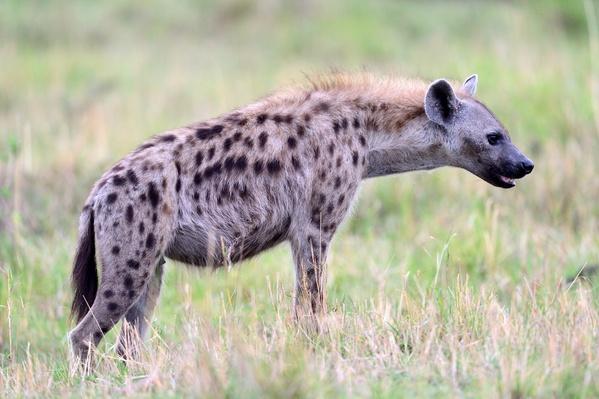The image is a detailed color photograph taken in a landscape orientation, showcasing a single animal—a hyena—positioned in the center of the frame. The hyena's figure dominates the photo, standing broadside and facing towards the right. The scene unfolds in the wilderness, with tall grass stretching out as far as the eye can see. The grass is a mix of light green with patches of off-colored beige, indicating dead grass scattered throughout.

The hyena has a distinctive appearance characterized by a light tan coat adorned with black spots that extend along its sides, back, and down to its legs. A blondish mane runs along the top of its neck, giving it a somewhat fierce and alert look. Its long snout, rounded ears, and sharp teeth, visible in its parted mouth, add to its predatory impression, alongside a piercing stare that looks ready to pounce. Its tail, covered in dark, long hair, hangs straight down.

The overall composition is sharp in the foreground, where the hyena stands, and fades slightly out of focus in the background, highlighting the realism and detail of the animal against the contrasting green and beige hues of the grassland.